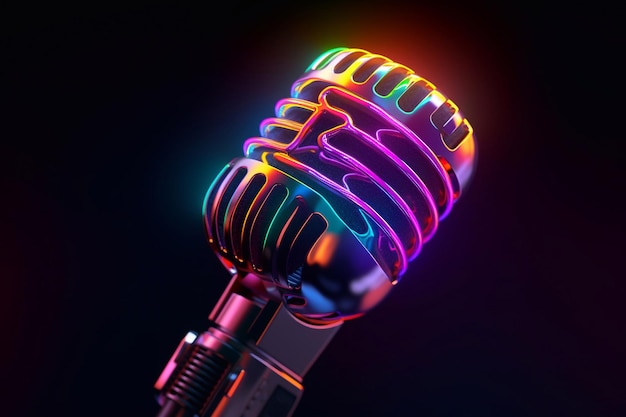This digital rendering features a vintage-style microphone reminiscent of those used by Elvis Presley, prominently displayed against a stark black background. The microphone is depicted in a highly detailed and colorful manner, with reflective rainbow hues gleaming off its metallic surface. The microphone's stem starts from the lower middle part of the image and extends diagonally to the upper right corner. 

Intricate cutouts are distributed across its surface: vertical slots at the base, horizontal slits in the middle, and more vertical openings near the top, precisely where one would speak into. The vivid colors transition across the microphone, starting with red and silver near the bottom. As the eye moves upward, lush shades of green, yellow, red, blue, purple, and orange intermingle, creating a captivating neon effect with bright lime green, blue, and lavender hues. This striking contrast against the black backdrop emphasizes the microphone's radiant and nostalgic aesthetic.